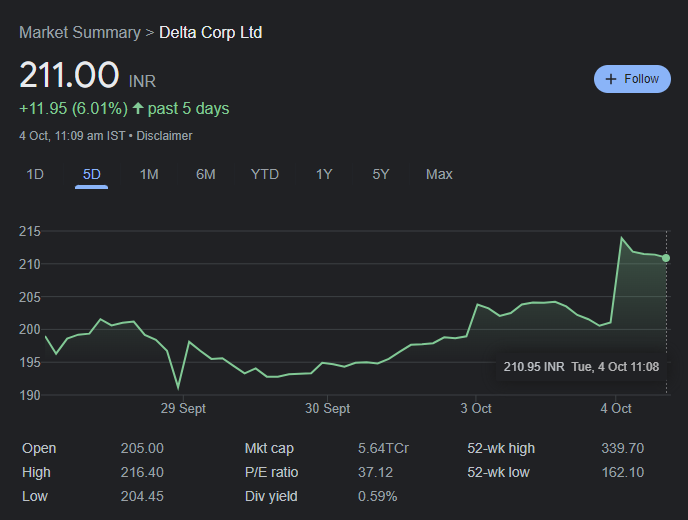The image displays a detailed market summary for Delta Corp Ltd. At the top of the page, the bold title "Market Summary" is prominently featured, followed by the company name "Delta Corp Ltd." Below this, the current stock price is displayed as "211.00 INR," with a notable increase indicated by "+11.95 (6.01%)" and an upward arrow denoting the positive change over the past five days.

Further details reveal that the last update was on "October 4th, 11:09 a.m. IST." Adjacent to this information, there is a conspicuous blue "Follow" button, suggesting that users can click it to receive updates about Delta Corp Ltd.

The graph occupies the central portion of the image, charting the stock's performance over the past five days. The X-axis spans from "September 29th" to "October 4th," while the Y-axis ranges from "190" to "215" in five-rupee increments. The line graph itself is green, contrasting against a black background. 

Below the graph's main area, detailed metrics include "Open: 205," "High: 216.40," "Low: 204.45," "Market Cap: 5.6 TCR," "P/E Ratio: 37.12," "Dividend Yield: 0.59," "52-Week High: 339.70," and "52-Week Low: 162.10." Additionally, there are various time-period options (1D, 5D, 1M, 6M, YTD, 1Y, 5Y, Max) displayed, with "5D" currently selected, providing a focused view of the recent stock performance.

Overall, this graphic provides a comprehensive view of Delta Corp Ltd.'s stock status, with key financial indicators and dynamic performance tracking over the selected timeframe.